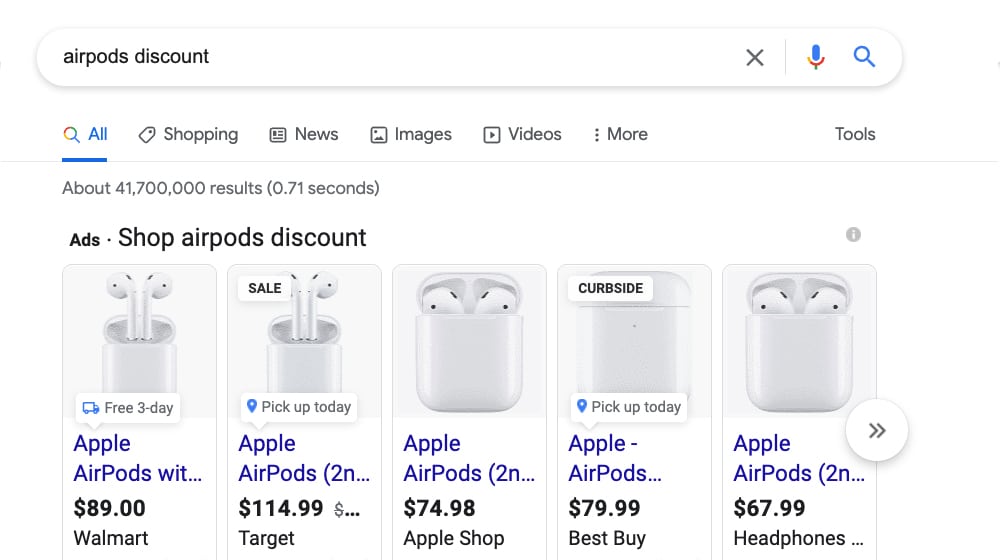The image depicts a results page from a Google search for "Airpods discount." At the top of the page, there is an oval-shaped rectangular Google search bar outlined in a gray-shaded box, but the interior is white. Inside the search bar, the query "Airpods discount" is displayed. On the right side of the bar, there are three icons: an X key to clear the search, a microphone for voice input, and a magnifying glass to initiate the search.

Below the search bar, there is a series of hyperlink drop-down menus allowing the user to refine various parts of the search. Following this, the search statistics are prominently displayed, indicating that the search term yielded approximately 42 million results in less than a second.

Under the search statistics, there are five thumbnail images accompanied by brief descriptions of AirPods. Each image shows a slightly different view of AirPods, and the accompanying text provides information on the store where each item is available and its respective price.